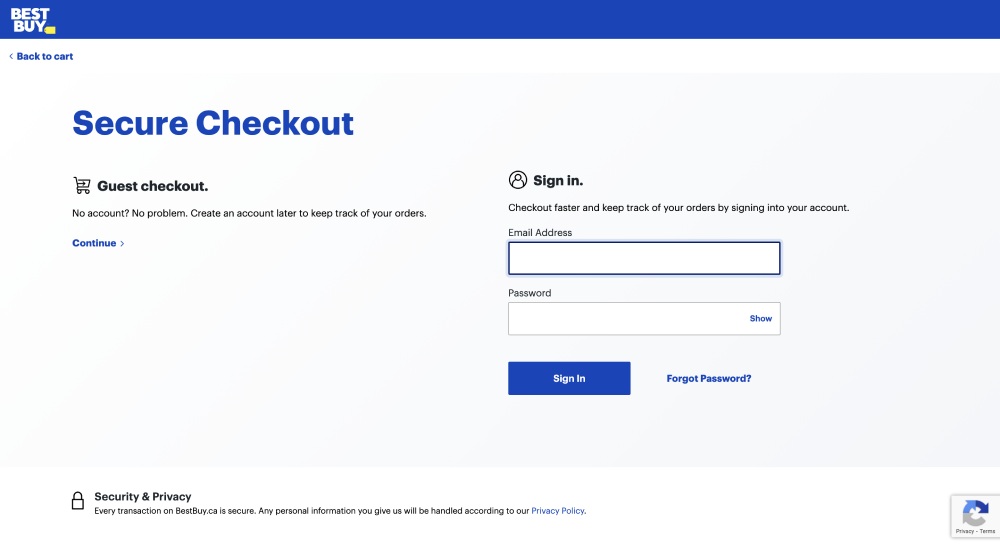The image depicts a Best Buy checkout page with a banner at the top. The top left corner features the iconic yellow price tag logo with "Best Buy" written in white against a blue bar that stretches the width of the header. 

Below the header, there is the text "Back to Cart," indicating an option to return to the shopping cart. The primary content of the page presents options for proceeding with a secure checkout. Users can choose between a guest checkout or signing in with an existing account. 

The sign-in section encourages users to "Check out faster and keep track of your orders," and includes fields for email and password. A "Forgot password?" link is available for those who need it. The sign-in process is initiated by clicking a blue button labeled "Sign in." 

The page emphasizes security and privacy, stating that all transactions are secure and personal information is managed according to Best Buy's privacy policy. This policy can be accessed via a blue hyperlink. To the right, there is an icon with a gray and blue revolving arrow, symbolizing terms of privacy and security.

The page's color scheme includes white text on a blue background for the Best Buy banner, blue buttons for "Sign in" and "Continue," and a light gray box around the secure checkout and sign-in area. The security and privacy text is displayed in white.